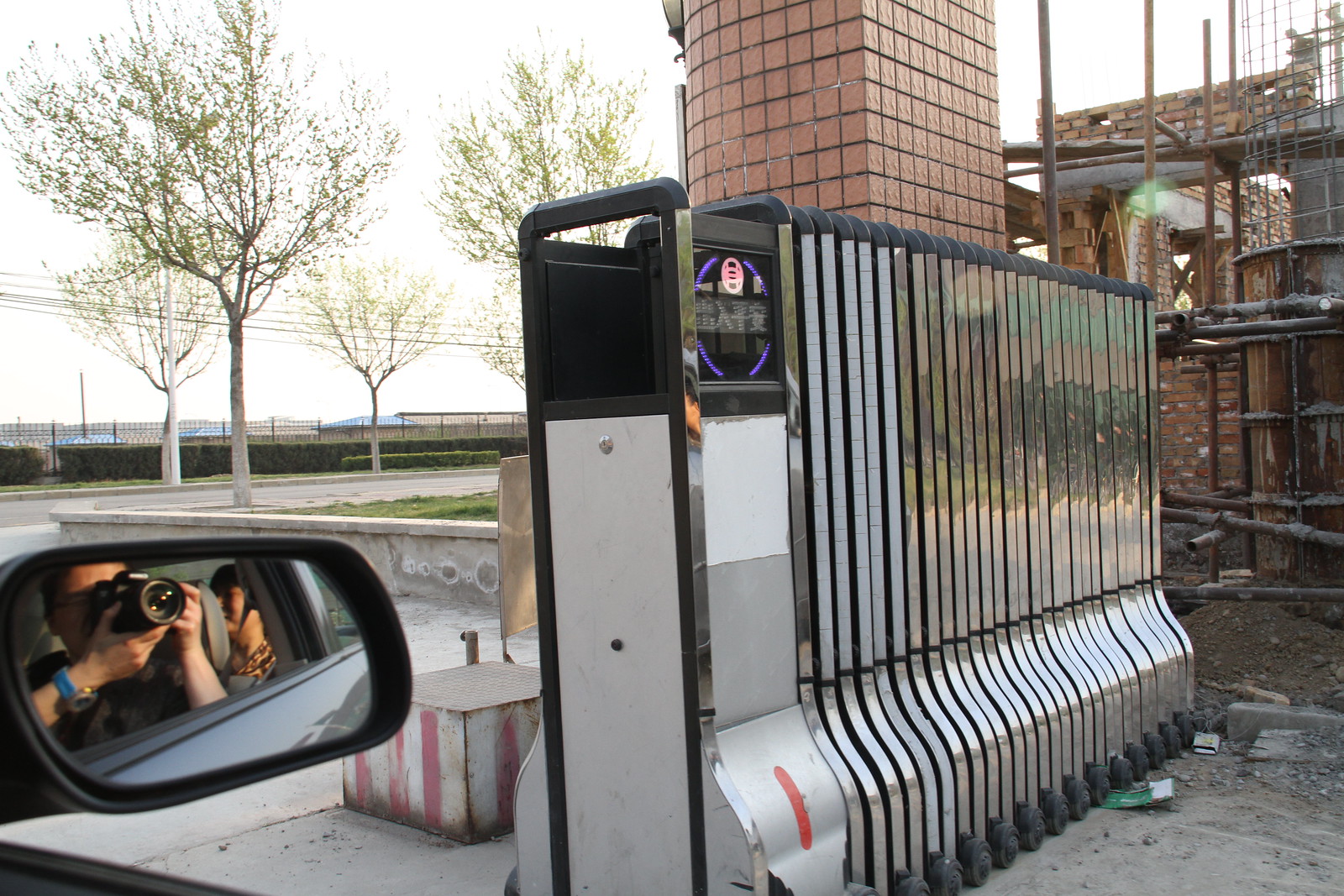In this daylight color photograph, a male with tan skin and dark hair is seen taking a picture through the window of a car from the front passenger seat. His reflection is visible in the car's side mirror, showing him holding a camera. Behind him, someone is seated in the backseat. The background reveals a worn cement landscape with sparse elements. On the right, there is a deteriorating brick building with scaffolding and a red brick wall, possibly with a window space. Adjacent to the street on the left, small planted trees and a hedge are visible. The central focus seems to be a long, rectangular structure with shiny metal bars, resembling a subway station entrance or a metal gate, atop what looks like a shelf. The sky is overcast, adding a grayish tone to the entire scene.